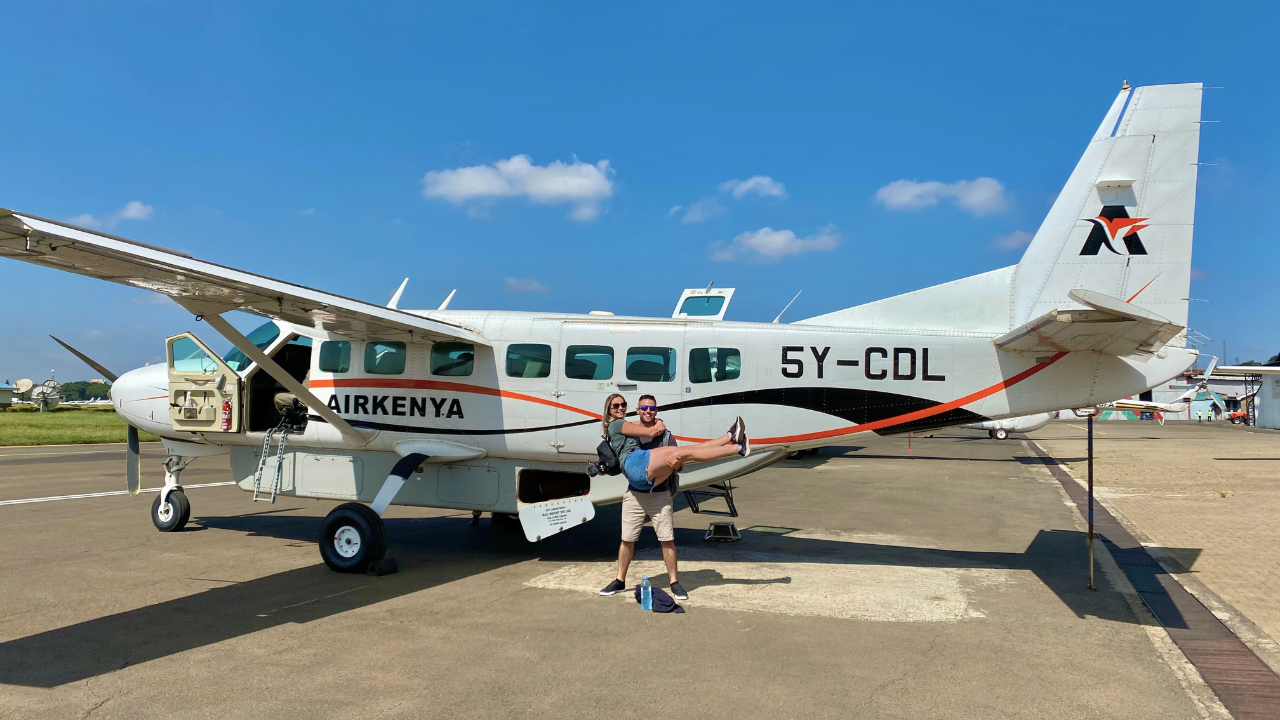A bright, clear day at a small airport sets the backdrop for a lively scene. In front of a white and black single-propeller Air Kenya plane, two people share a playful moment. The aircraft features both an orange and a black curved stripe, intertwining across its exterior, with the registration number 5Y-CDL labeled clearly on the tail end and an 'A' marking on the tail. The plane boasts seven windows on its passenger side. A man, dressed in khaki shorts and sunglasses, energetically lifts a woman clad in jean shorts, a t-shirt, sunglasses, and a backpack. She wraps her arms around his neck as he supports her. In front of them, a jacket and a water bottle lay on the tarmac. The scene is set against a backdrop of green grass to the left, a cluster of white satellite dishes to the right, and a sky adorned with a few scattered clouds, capturing the essence of an impending journey.